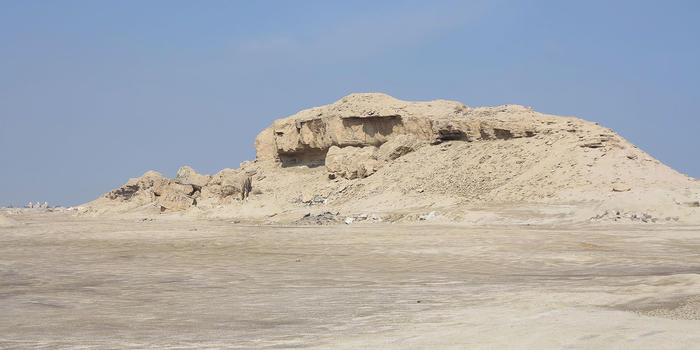The image depicts a vast desert landscape dominated by a large, imposing natural rock formation. This rugged, beige-colored structure, adorned with shadows that cast a darker brown hue, stands prominently in the center-right of the photograph. The formation features cliffs and overhangs that taper down to the left side. The surrounding sandy terrain is a light tan color, typical of desert sands, and almost forms a hill around the base of the rock. Adding to the desolate atmosphere, the environment is largely barren, with only two cacti visible at the base of the rock formation. In the distance, faint outlines of buildings suggest the scale of the formation, indicating it is much larger than it initially appears. The sky above is a clear pale blue, with minimal cloud cover, enhancing the stark, arid feeling of the scene. The ground between the photographer and the rock formation appears dark, possibly indicating moisture, though no water is seen. This isolated and starkly beautiful location resembles a place people might visit for specific activities like caving, rather than a typical vacation destination.